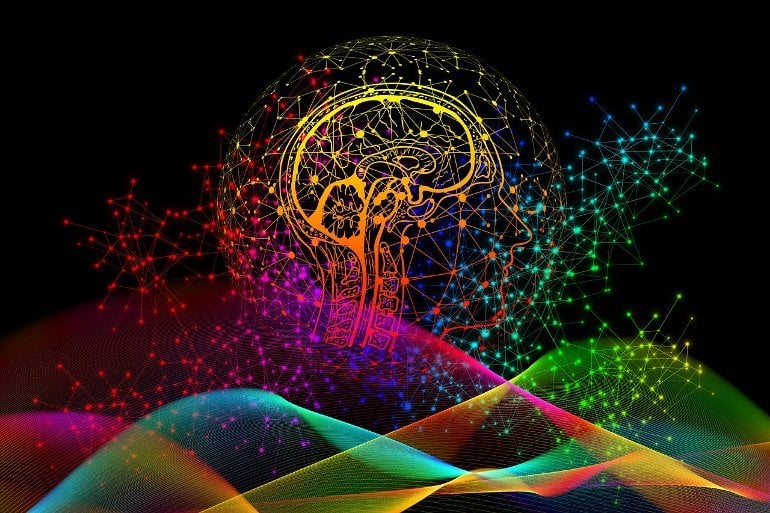This digital artwork features a captivating and psychedelic depiction of a human profile, viewed from the side, with a focus on the brain and upper spinal cord presented in a wireframe model. The background is solid, matte black, creating a stark contrast that highlights the vivid, cascading rainbow lines forming hill-like shapes at the bottom of the image. These lines, in shades of magenta, cyan, teal, orange, and green, give the impression of colorful, undulating sand dunes. Above these dunes, there is an intricate network resembling a spider web, crisscrossed with digital needle-like structures that appear to have glowing orbs at their ends in colors such as green, blue, orange, pink, and yellow. Surrounding the head is a sphere, further adorned with constellation-like patterns and interconnected lines, adding a sense of cosmic exploration. The artwork conveys themes of mind expansion and digital complexity, offering a visually stimulating experience that might serve well as a computer wallpaper.